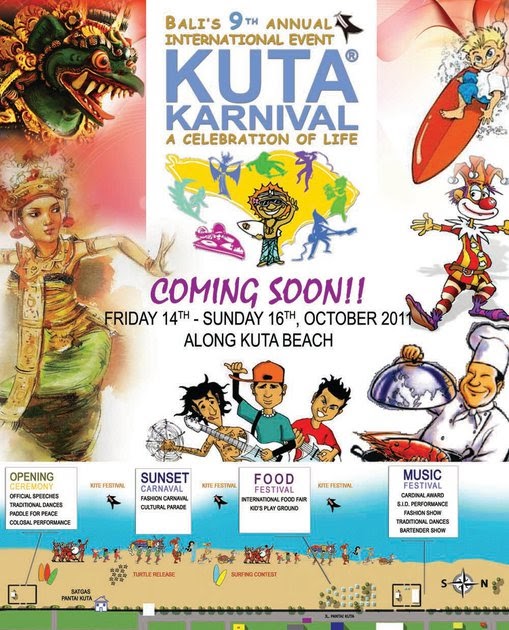The advertisement is a vibrant and visually striking poster for the 9th annual Kuta Carnival, also known as the Celebration of Life, held in Bali. The event is scheduled to take place from Friday, October 14th to Sunday, October 16th, 2011, along Kuta Beach. The poster features a mix of colorful illustrations and different artistic styles, including an oriental dragon in the top left corner and a classical Indian dancer below it. The top right corner showcases a cartoon character surfboarding, with a cartoon clown below him. Further down, there is an image of a chef presenting a lobster on a plate, flanked by three cartoon characters in a band to his left. The text includes key details such as "KUTA Carnival" in blue and "A Celebration of Life" in gold, as well as mentions of various attractions like the opening ceremony at sunset, a carnival food festival, and a music festival. Overall, the poster conveys the festive and diverse spirit of the Kuta Carnival through its dynamic visual elements and comprehensive event information.